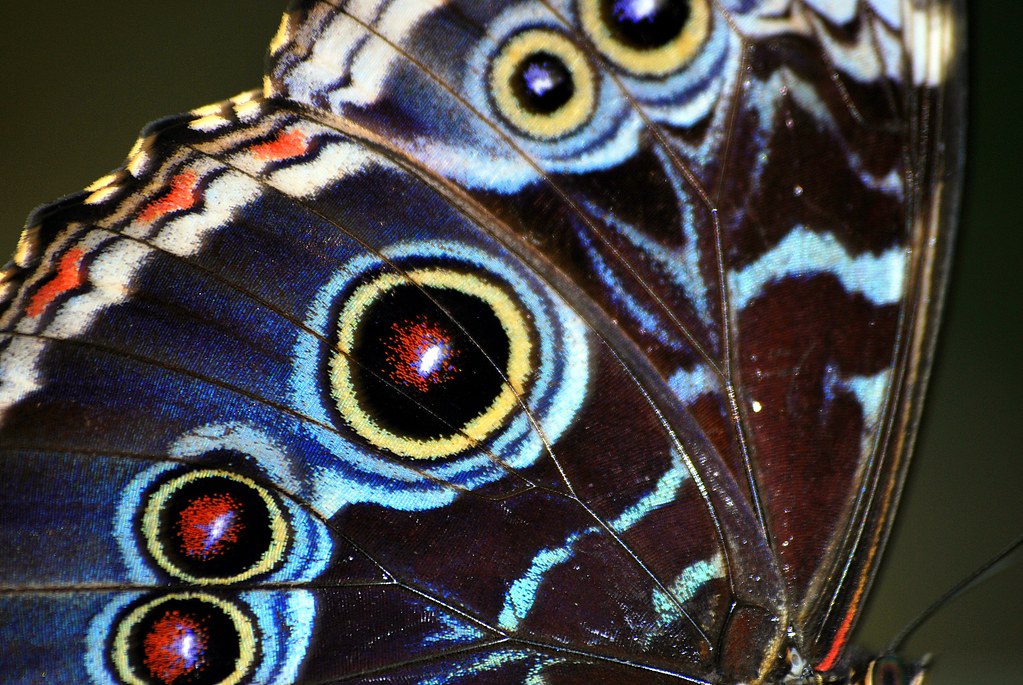This is a detailed close-up photograph of a butterfly wing, showcasing a mesmerizing blend of intricate patterns and vibrant colors. The backdrop of the wing is predominantly dark, featuring deep tones of black and navy blue. One can barely make out a portion of the butterfly's head or antenna at the bottom right, adding a subtle, elusive detail to the composition. The wing itself is adorned with a series of striking, curvaceous lines and circles that align diagonally across its surface. The outermost lines are dark with white specks, followed by curves of brown, white, and a striking orange design. The wing's most captivating feature is the large, concentric circles. These start with an outer light blue ring, inside of which lies a black circle, followed by a yellow ring, and then a central dark black splotch. Within this black area are red specks and a final white dot at the very center. These circles, appearing to mimic eyes, likely serve as a defense mechanism against predators. Additionally, the top portion of the wing showcases undulating lines of white and light blue, incorporating smaller circles with yellow, black, and blue centers. The entire wing is detailed with hints of orange, red, and yellow along its edges, creating a visually stunning and complex pattern.